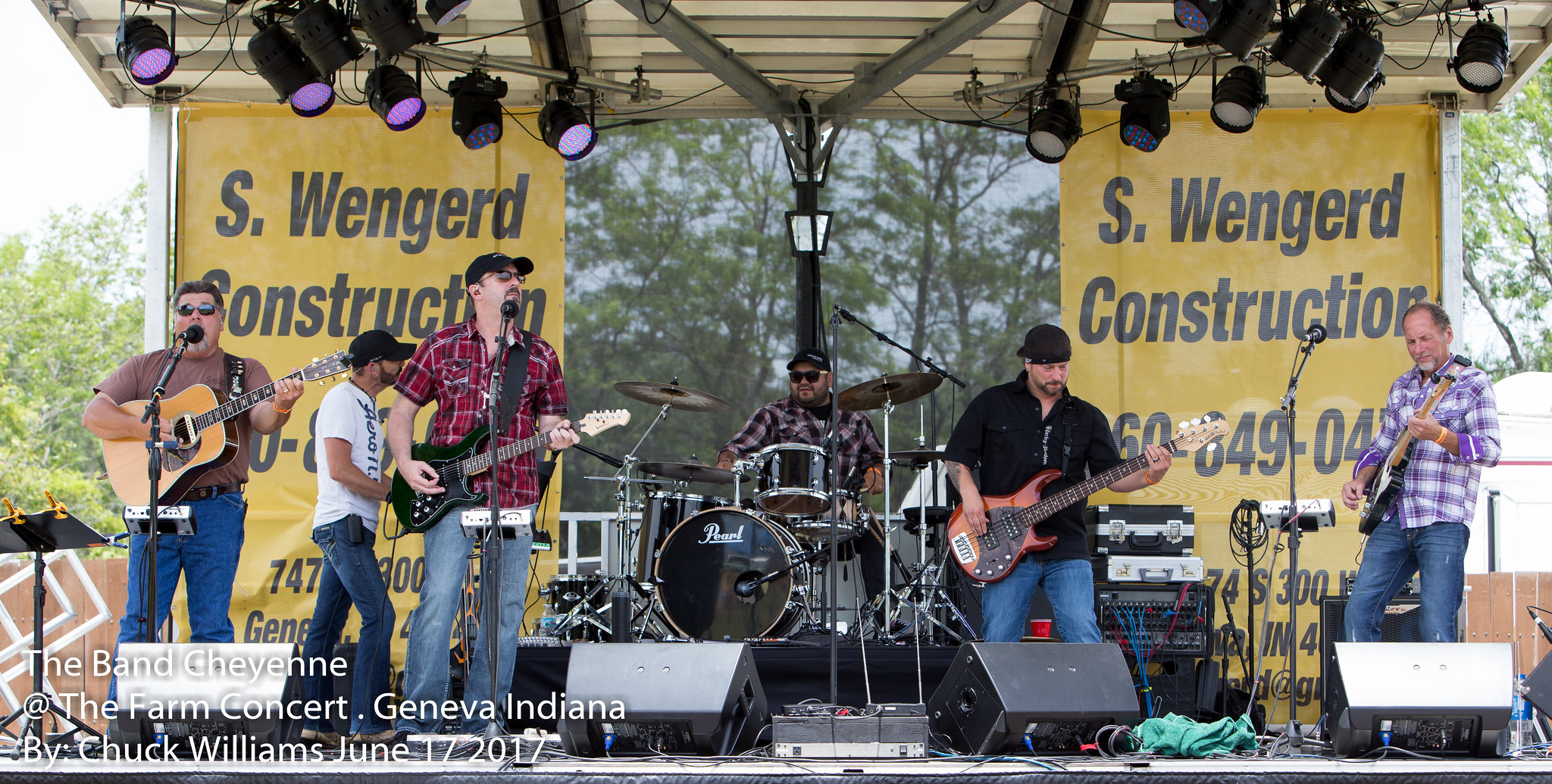The image captures an outdoor musical concert, set against a backdrop of clear skies and lush trees, suggesting a daytime event. The stage, equipped with a ceiling fitted with multiple lights, reveals a lively scene with six band members performing. On both sides of the stage, yellow banners display an advertisement for "S. Wengert Construction," accompanied by the phone number 606-484-9049. 

From left to right, the first musician is an elderly man with a white French beard, black hair, and black glasses. He is wearing a brown t-shirt and blue jeans, playing a guitar, and singing into a microphone. Next, a man in a black cap, white t-shirt, blue jeans, and a beard walks across the stage. The third member, another guitarist, stands at a mic with an electric guitar. He sports a black cap, sunglasses, a red checkered half-shirt, blue jeans, and a French beard. Behind him is the drummer, identifiable by his black cap, sunglasses, and checkered shirt.

The next guitarist wears a black cap, black half-shirt, blue jeans, and displays heavily tattooed arms. Finally, an older man stands on the far right, with a white French beard and balding hair, clad in blue jeans and a purple-and-white checkered shirt, playing a guitar with a microphone in front of him. Scattered across the stage are various instruments, speakers, boxes, and wires, adding to the authentic concert atmosphere. In the bottom left corner of the image, the text reads: "The band Shane and the Farm, Concert, Geneva, Indiana, by Chuck Williams, June 17, 2017."